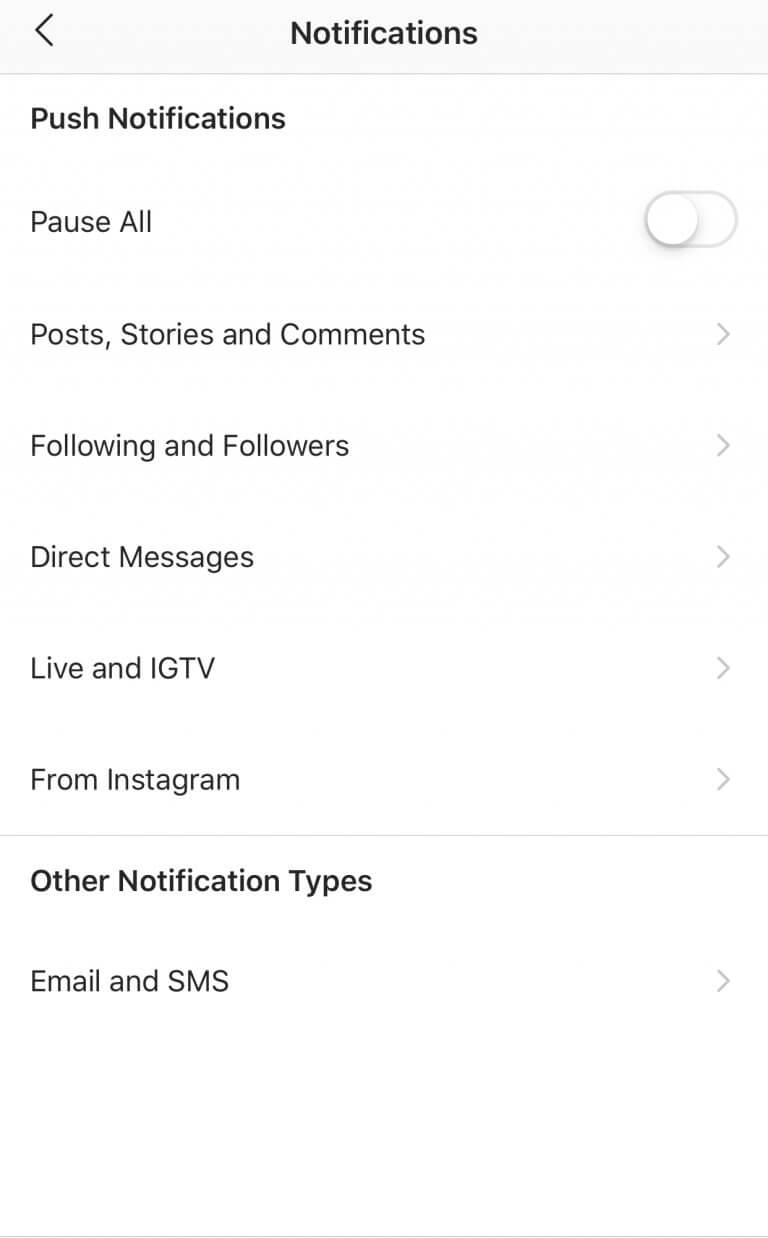In the image, we see a notification settings window presented in a clean and minimalist black and white design. At the top, there is a "Notifications" heading in its own distinct bar, followed by a separator line. Below this line, the first section is titled "Push Notifications" in bold, offering a range of customizable options.

The first option in this section is "Pause All," allowing users to temporarily halt all notifications. Moving down, the subsequent options are listed in order: "Posts, Stories and Comments," "Following and Followers," "Direct Messages," "Live and IGTV," and "From Instagram."

A separate section below these, marked by another bold heading "Other Notification Types," includes further settings with "Email and SMS" being the primary option listed. The entire window is displayed in white mode, featuring a white background with black text, ensuring high readability. At the top of the screen, within the notifications bar, there is an arrow icon for navigating back, maintaining the window's straightforward and user-friendly design.